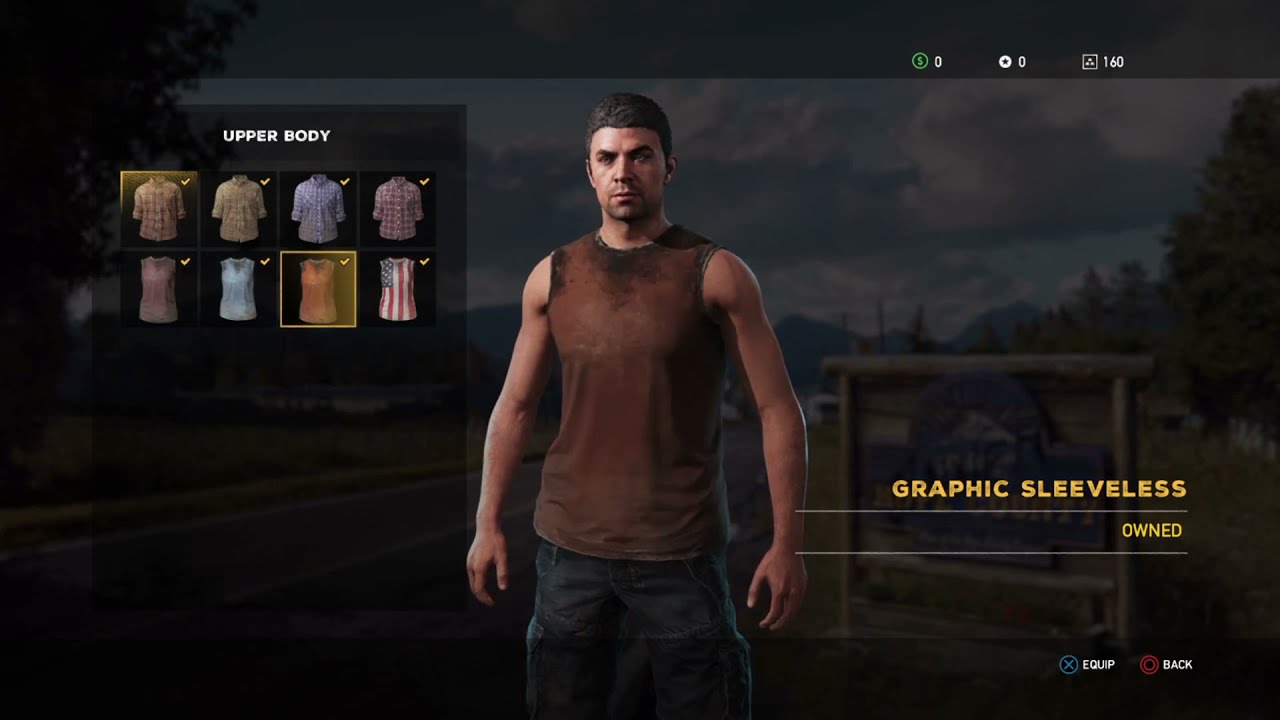The image is a detailed screenshot of a video game character customization menu. At the center, a realistic-looking white male character with tight black hair is standing straight and facing the camera. He sports a serious expression while wearing a brown sleeveless t-shirt and blackish denim cargo pants. His arms are hanging at his sides. The background portrays a dark, outdoor farm-like environment under a cloudy blue sky, with mountains and a faded sign possibly indicating a city entrance in the distance, framed by trees.

On the left side of the screen, there is a menu displaying options for different upper body clothing, including both short-sleeved and sleeveless shirts. An image of the currently selected shirt, which matches what the character is wearing, appears in the upper left, under a section labeled "Upper Body." 

On the right side, text indicating the shirt's attributes reads "Graphic Sleeveless," followed by the word "Owned." Below this text are two buttons, "Equip" and "Back," suggesting options for the player to modify the character's attire.